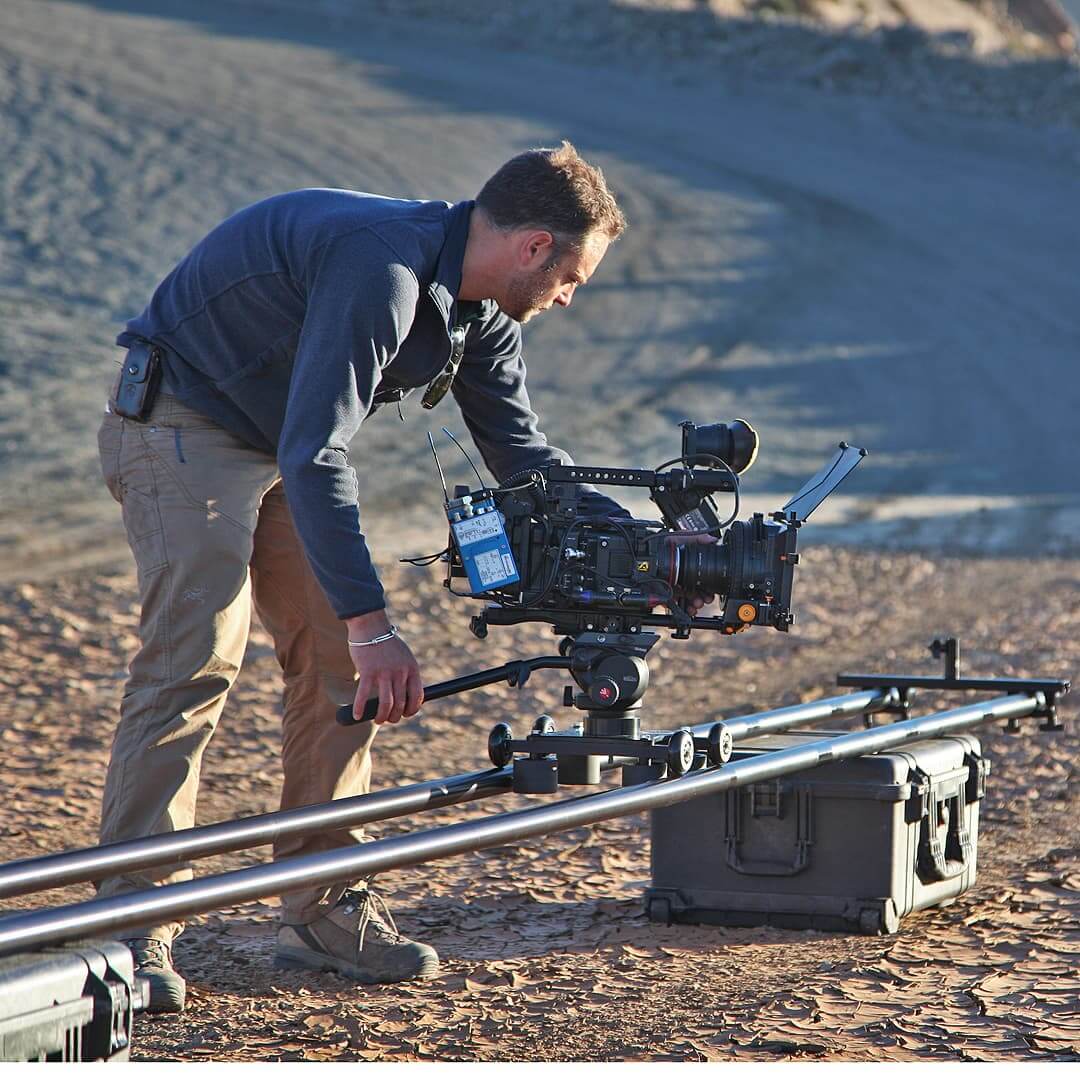In this outdoor photograph, a detailed scene unfolds centered around a professional film setup. Dominating the middle of the image, a large black camera designed for movie or commercial filming is securely mounted on a wheeled dolly. The dolly glides on twin metal rails, which run diagonally from the lower left to the upper right of the frame. Supporting these rails are dark-colored, plastic suitcase-style boxes. Operating the camera is a man fully engrossed in his task; he is bending over with meticulous focus. His attire includes a long sleeve blue jacket, with sunglasses tucked at the center, tan pants, and brown shoes. Additionally, he has a cell phone holder clipped to his pants and wears a bracelet. His right hand steadies the camera handle, ensuring precise tilts, while his left hand is positioned behind the camera. The dry, flaky dirt ground and an arcing dirt road in the background add to the rugged outdoor setting. The careful setup suggests they are in the process of filming a smooth, moving shot, vital for capturing dynamic footage without jerky motions.